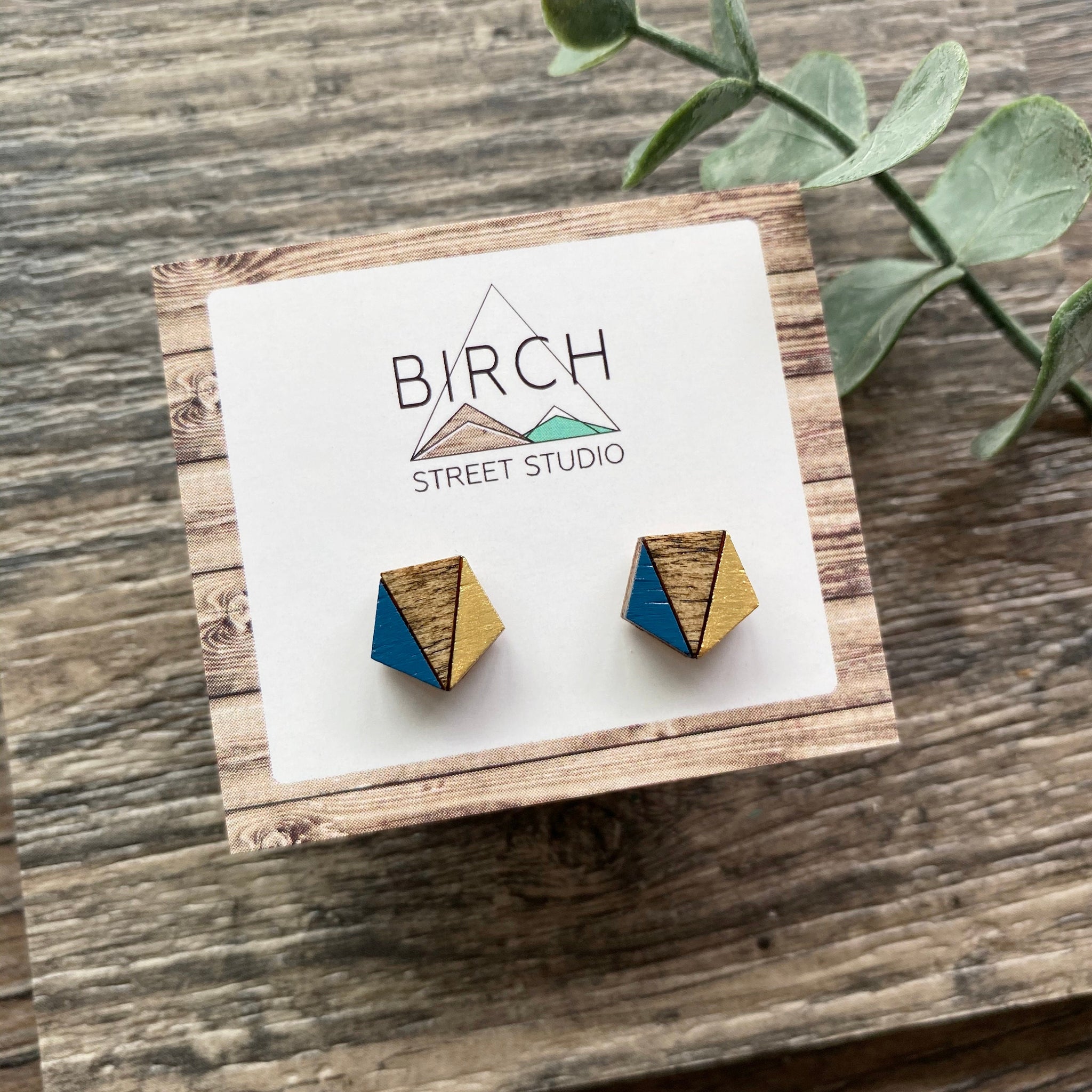This meticulously composed photographic image features the top view of a wooden box resting on a wooden tabletop characterized by various shades of brown, from light to dark. The box is square and made of light brown wood, accentuated by a white label that mirrors its shape. Central to the composition, the label prominently displays the logo of Birch Street Studio, which includes the text "Birch Street Studio" and a graphic of a triangle encapsulating two mountains—one brown and the other green with a white peak.

Enhancing the visual interest, the top right corner of the image includes a sprig of eucalyptus with soft green leaves, adding a natural touch to the setting. Set against this backdrop, the box is oriented at a slight angle, leaning upward from right to left. Below the logo on the label are two uniquely designed stud earrings resembling triangles. Each earring, composed of an inverted triangle flanked by two right-side-up triangles, features a combination of colors—including shades of blue, yellow, and what appears to be gold—creating a hexagonal appearance. These earrings could also be interpreted as miniature triangular sculptures, adding a functional artistic element to the composition. The entire scene is captured within a square frame, creating a visually clean and cohesive product shot.